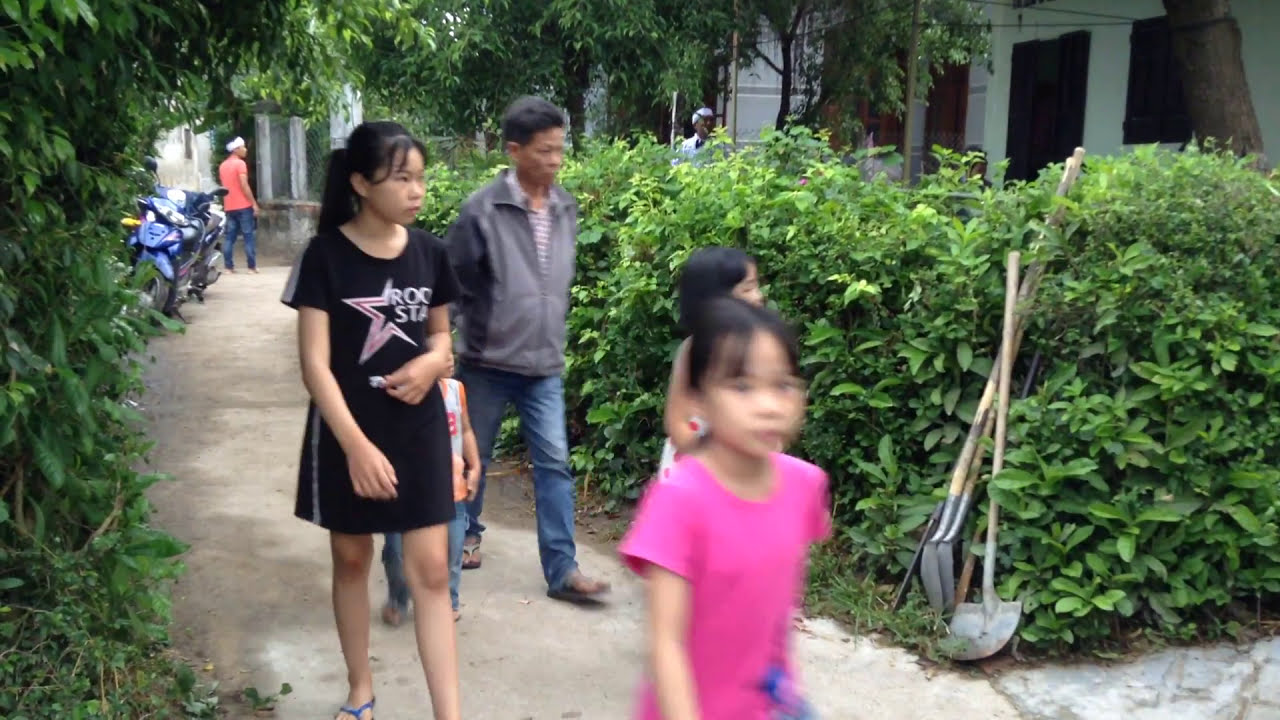This image captures a detailed scene of a family of five, likely of Asian descent, strolling together down a sidewalk lined with bushes near some buildings. At the forefront is a little girl, approximately seven years old, wearing a bright pink shirt and black hair possibly accented with glasses, though her face is slightly blurred. Right behind her is another young girl, with visible black hair, wearing a white dress adorned with red polka dots. On her left is an older girl, around 13 or 14, dressed in a black 'Rock Star' t-shirt and a black skirt with a gray stripe. She has shoulder-length black hair styled in pigtails and is wearing blue flip-flops. Walking just behind these girls is a young boy in a sleeveless white shirt and blue jeans, alongside a man in a gray jacket with black sleeves, also in blue jeans, who appears to be their father. In the distant background, another man wearing a pink or orange shirt and black shoes can be seen near a few motorcycles. The path they are walking on is bordered by an array of shovels and possibly other gardening tools resting upright at a slight angle against the bushes. The lush greenery around adds a vibrant natural backdrop suggesting a serene environment.